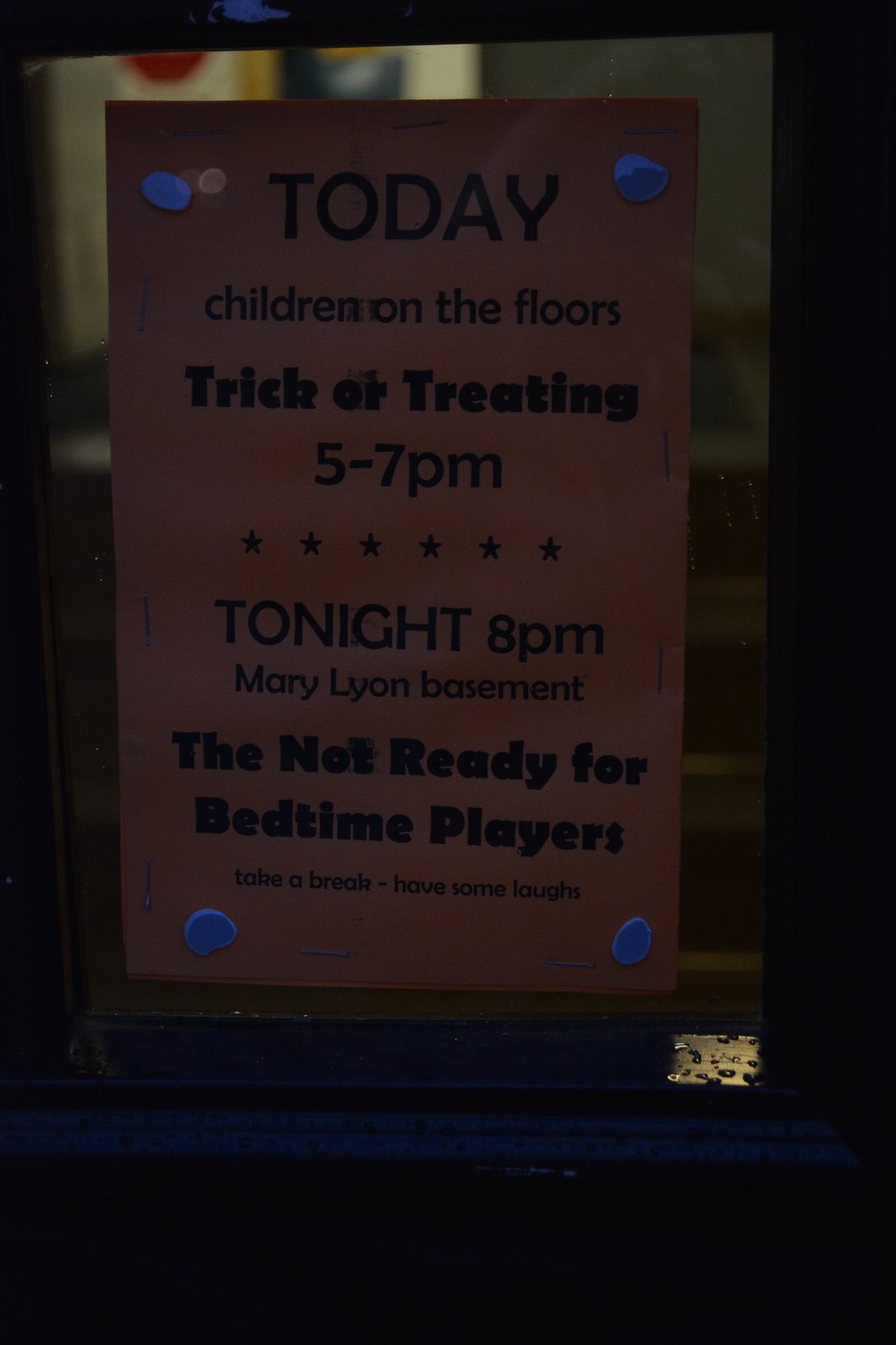The image depicts a darkened photograph of a poster adhered to a window, possibly a door with a visible frame, as water droplets suggest it's been raining outside. The poster, appearing to be either orange, pink, or red, is affixed to the window using four light blue adhesive dots, one in each corner. The text on the poster, written in black ink, announces: "Today, children on the floors trick-or-treating, 5 to 7 p.m. Tonight, 8 p.m., Mary in Lyon basement, the not-ready-for-bedtime players. Take a break, have some laughs." A line of six stars separates the two announcements. The background of the image reveals a blurred interior, indicating the photo was taken from inside a building.